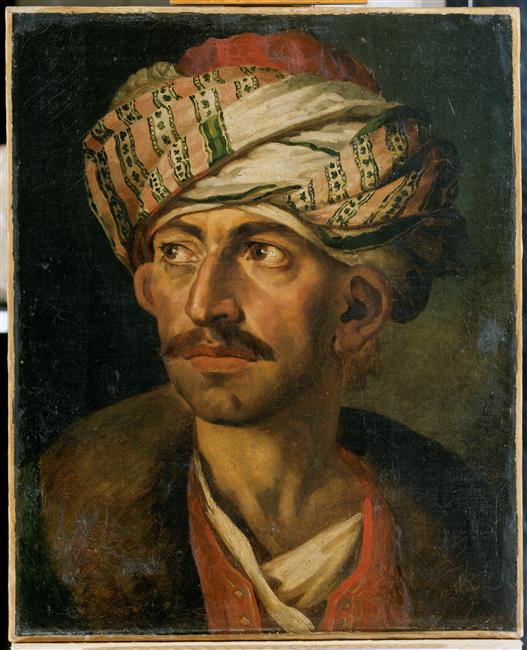This is a vertically aligned, rectangular portrait painting of a Middle Eastern or potentially Central Asian man adorned in a distinctive, ornate headdress. The turban, intricately wrapped around his head, showcases a mix of colors and patterns: gold with green and beige designs, a striking red center, and decorative white and green stripes. His ears, partially bent forward due to the wrap, peek out from beneath the headdress. The man has brown eyes and eyebrows, a closely cropped brown mustache, and a serious expression as he gazes off to the left. His slightly furrowed brow and closed lips add to his contemplative demeanor. He is dressed in a layered outfit consisting of a white shirt, a red shirt adorned with gold buttons, and a heavy brown fur jacket or coat with an open red vest. The painting is framed with a light brown border, and the background is a dark blend of black and brownish-green hues, enhancing the subject's presence and solemn expression.